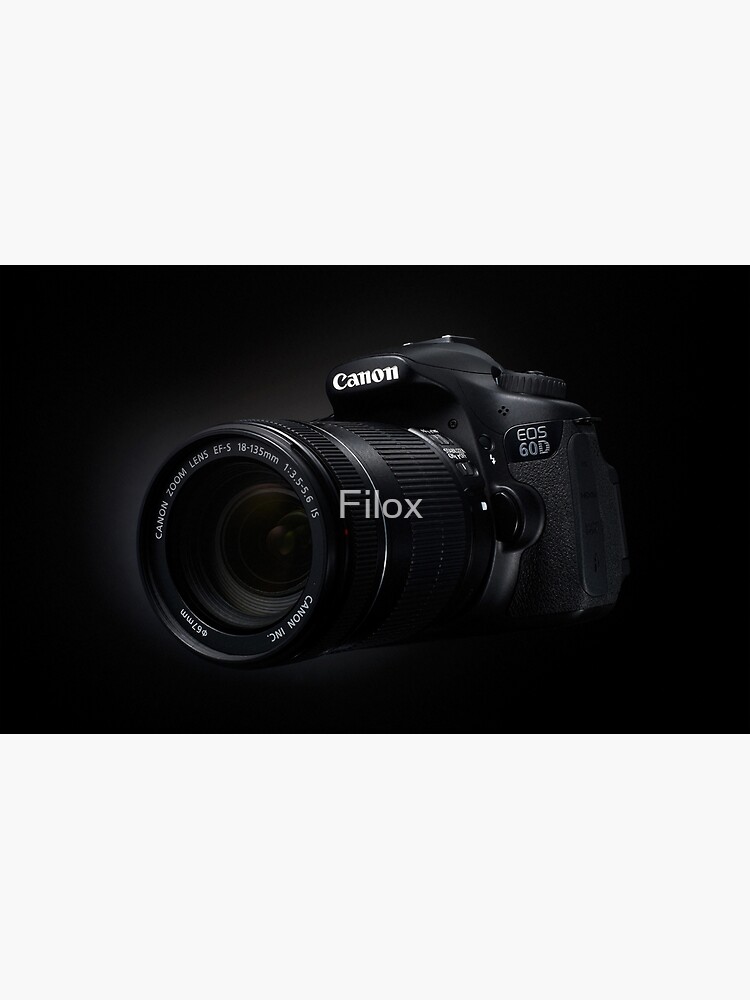This is a color photograph in landscape orientation showcasing a black Canon EOS 60D camera set against a black background, making the camera's details subtly highlighted by gray illumination along the sides. The Canon logo in white is prominently displayed near the top of the camera body. The camera features a substantial zoom lens, which occupies a significant portion of the visible image. The lens is imprinted with the text "Canon Zoom Lens EF-S 18-135mm 1:3.5-5.6 IS" and "67mm." Adding to the composition is a gray watermark that reads "Phylox," overlaying the camera. The photograph employs a representational realism style, emphasizing detailed visual accuracy.